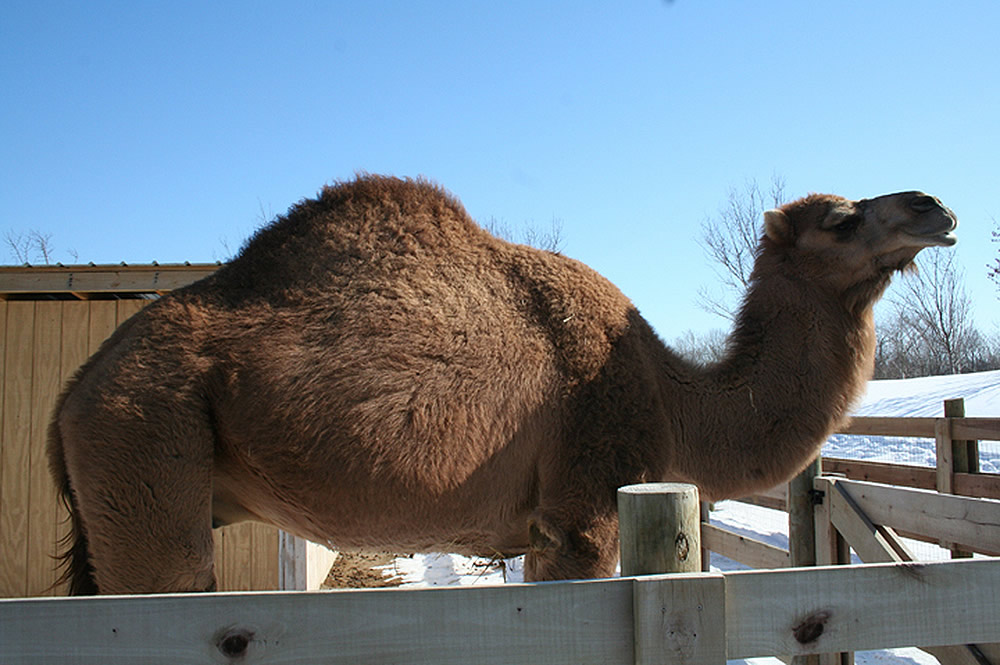This landscape-oriented color photograph captures a bright, sunny winter day with a clear blue sky. The ground is covered in snow, reflecting the frigid temperature of the scene. Centered in the image is a large, tall camel with short brown fur and a single, medium-sized hump on its back. The camel is standing in profile, facing to the right, with its head held high and its neck arched gracefully. A slight black mane crests its neck, and it has a black tail. The camel stands inside a fenced corral made of light wooden paneling attached to round wood poles, which come up to about half its height. Behind the camel, on the left side of the photograph, there is a small, flat-roofed wooden building likely used for storage or as a shelter. The background features a line of barren, leafless trees standing against the deep blue horizon, further accentuating the wintry, cold atmosphere of the setting. Shadows cast by the bright sun create a striking contrast, enhancing the overall detail and realism of the image.